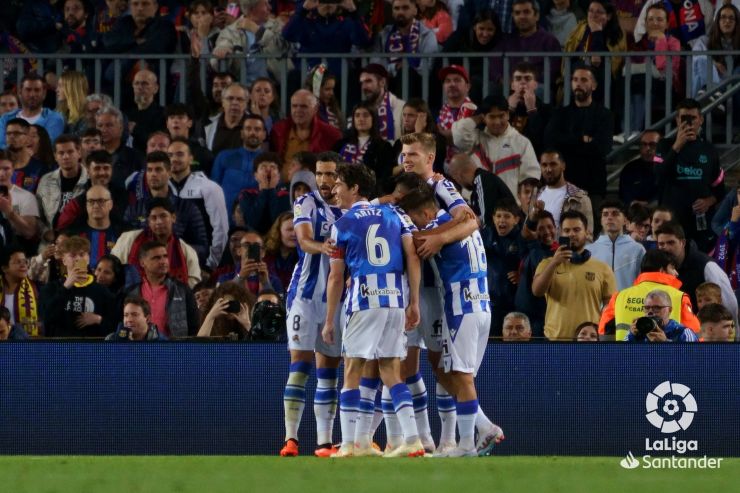In this vibrant photograph of a soccer game, about four to five players, donned in blue and white striped jerseys with white shorts, are huddled together in a circle, looking off to the left side of the image and smiling. Prominently, the back of a player named Arte Aritz, wearing the number 6, is visible at the center, while another player's jersey displaying either the number 18 or 78 is to his right. All players sport white and blue socks with distinct orange cleats adding a pop of color. Surrounding them, the lush green field sets the stage, complemented by a bustling crowd behind a dark blue barricade. Fans from diverse backgrounds, including those capturing the moment with their cell phones, fill the audience section. The bottom right corner of the image features the La Liga Santander logo, framed by a circular icon, grounding this lively scene in a professional setting.